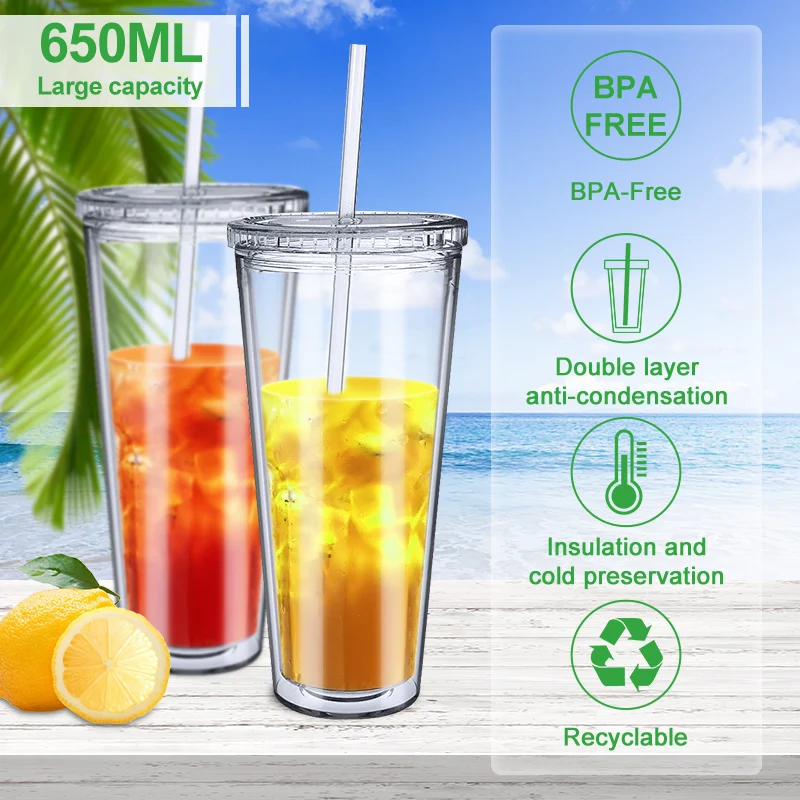This advertisement for BPA-free plastic cups showcases two clear, double-layered insulated cups, each with a straw, positioned on a wooden platform. One cup contains red juice while the other holds yellow juice, and both are topped with caps. The upper left corner highlights the cups' 650 ml large capacity in green writing on a white box. To the left of the cups, a whole lemon and a sliced lemon are displayed, accompanied by a palm leaf. The background features a serene blue sky with white clouds, overlooking the ocean. On the right, a box emphasizes the cups' features with green text in various circles: BPA-free (mentioned twice), a graphic of the cup with a straw, double layer anti-condensation, insulation and cold preservation, and a recyclable symbol. This image showcases these plastic cups as ideal for summer use, keeping your drinks cool and refreshing.